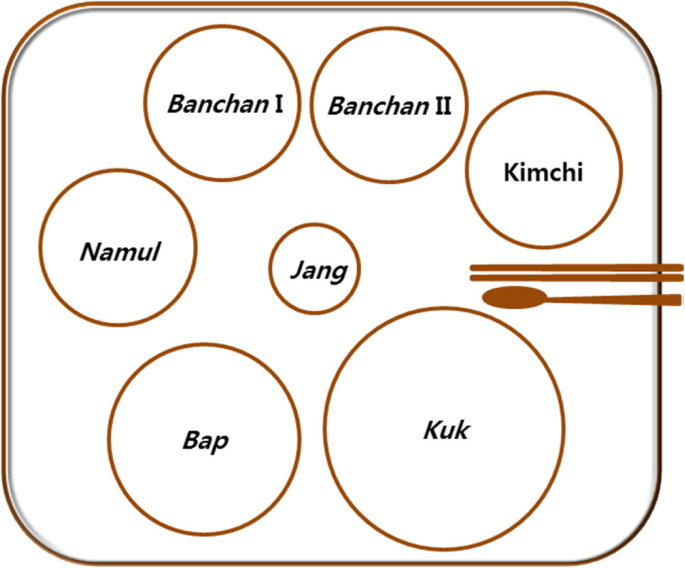The image depicts a computer-animated rectangular tray with rounded corners and a brown gradient outline, darker at the bottom right and lighter at the top left. Inset into the tray are seven white circles with brown outlines and black text labels. Starting from the top left, the circles are labeled "namul," "banchan 1," "banchan 2," and "kimchi." At the center is a smaller circle labeled "jang." Positioned at the bottom left is a slightly larger circle labeled "bap," and to its right, the largest circle labeled "kuk." To the right side of the tray, there is a pair of horizontal brown chopsticks and a brown spoon. The background of the image is white, complementing the brown tones of the tray and utensils. There is also a subtle shadow around the interior perimeter of the tray, enhancing its three-dimensional appearance.